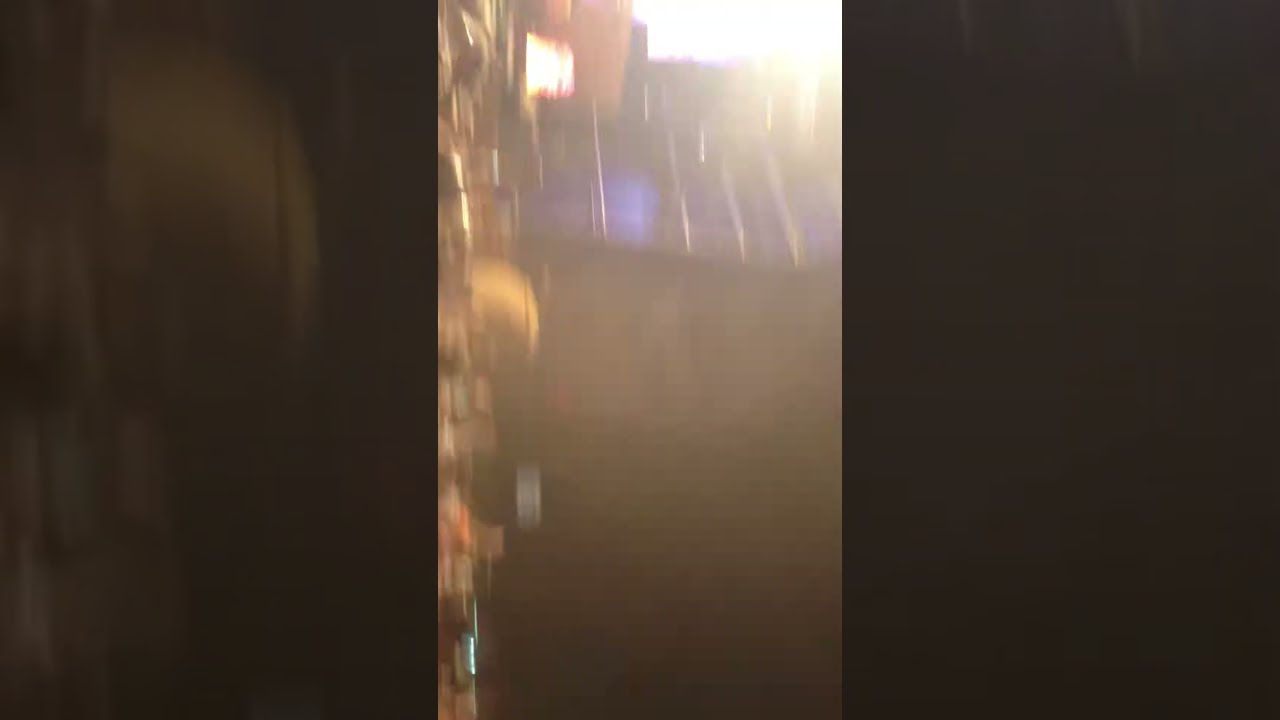The image is a blurry, rectangular photograph segmented into three vertical sections. The left and right sections form darker borders around the central image, which is visibly brighter, creating a noticeable contrast. The main central section appears over-illuminated, possibly due to a bright sun shining from the top right, adding to the blurriness and making it difficult to discern clear details. The color theme spans black, blue, and yellow, with occasional flashes of orange. Vague shapes within the center image suggest it may depict a scene along a road bordered by buildings, interspersed with glimpses of people and vehicles. The overall effect of the image is further amplified by glare and flash, rendering most elements indistinct and challenging to interpret.